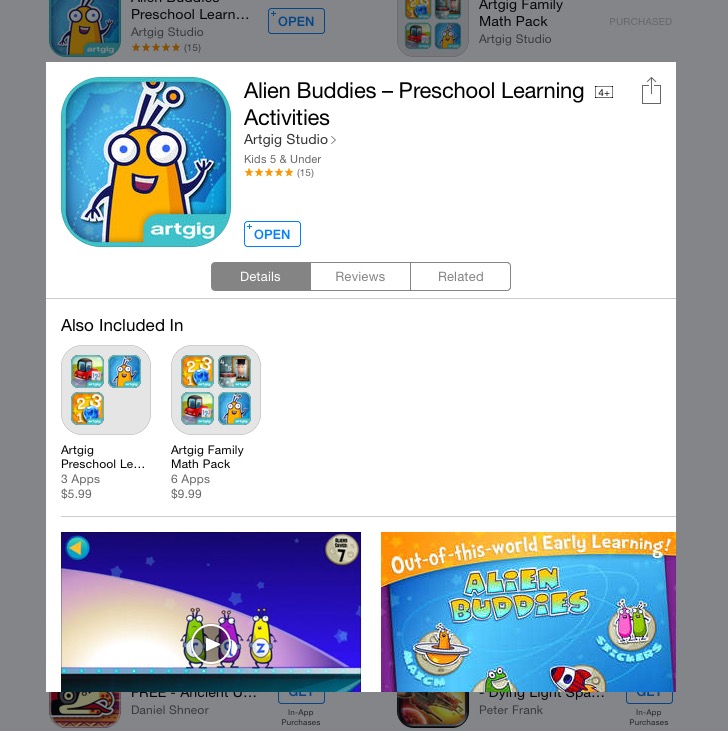The image depicts an app store interface featuring a highlighted app. 

A dark gray border surrounds the outside of the window, framing the central pop-up. The pop-up, set against a clean white background, showcases an educational app for preschoolers titled "Alien Buddies: Preschool Learning Activities" by Art Gig Studio. The app is specifically designed for children aged five and under and has received high praise, with a perfect five-star rating based on 15 reviews. 

In the upper right corner, there is a download icon. Adjacent to this, in bold black text, the app's title and details are listed. A prominent white button with blue text invites users to "Open" the app, while additional gray buttons labeled "Details," "Reviews," and "Related" offer further navigation options. The "Details" button is styled with white font on a gray background, whereas the other two buttons feature gray font on a white background.

Central to the pop-up is an image of the app's mascot: a charming, yellow alien with large, expressive eyes sporting blue pupils. The alien, characterized by its welcoming wave and antennae topped with orange tips, stands against a vibrant blue-green border. The backdrop prominently displays "Art Gig" in white text.

Below this scene, a promotional section highlights that the app is part of the "Art Gig Preschool Learning" series and the "Art Gig Family Math Pack," offering additional app bundles priced at $5.99 for three apps or $9.99 for six apps. The section includes a video and a screenshot of the app in action. The screenshot carries the text "Out of This World - Earth We Learning - Alien Buddies."